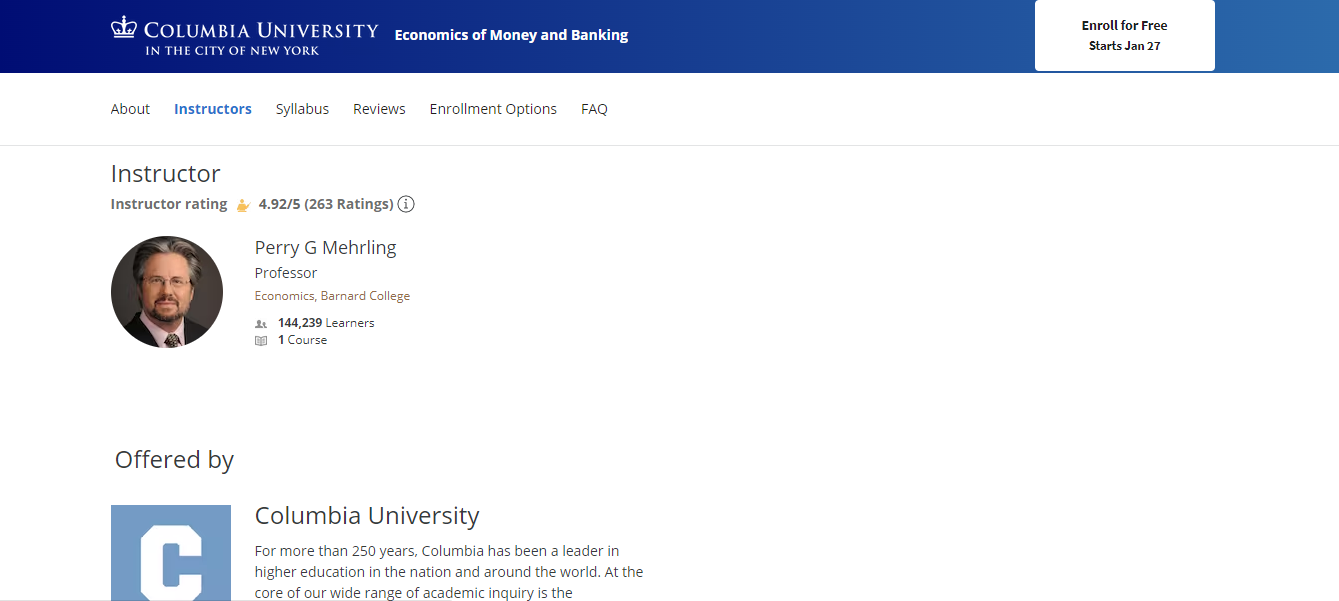The webpage is an instructor profile for Columbia University. At the top, there's a prominent blue bar featuring the university's iconic white crown symbol. To the right of the crown, "Columbia University in the City of New York" is displayed in white text. Directly below, in bold white text, the course title "Economics of Money and Banking" is prominently featured. On the far right is a white box with black text stating "Enroll for free starts January 27."

Beneath the blue bar, there's a navigation menu listing options: About, Instructors, Syllabus, Reviews, Enrollment Options, and FAQ. Currently, the focus is on the "Instructors" section. Here, we see the instructor’s profile with the following detailed information:

- Instructor Rating: 4.92 out of 5 (based on 263 ratings)
- Name: Perry G. Mehrling
- Position: Professor of Economics at Barnard College
- Teaching Experience: Perry has taught 144,239 learners and is associated with one course.
- Visual Description: Perry G. Mehrling is depicted wearing a pink shirt paired with a brown tie and a brown jacket. He also sports glasses, a goatee, and salt-and-pepper hair.

Below his picture, the section titled "Offered by" features the Columbia University logo—a white crown on a blue background—with the text "Columbia University." It emphasizes Columbia's 250-year legacy as a leader in higher education, known for a broad spectrum of academic pursuits. The text begins to explain the core principles of the university, but it cuts off before completion.

This detailed description aims to provide a comprehensive overview of the instructor profile page, highlighting key visual and textual elements.